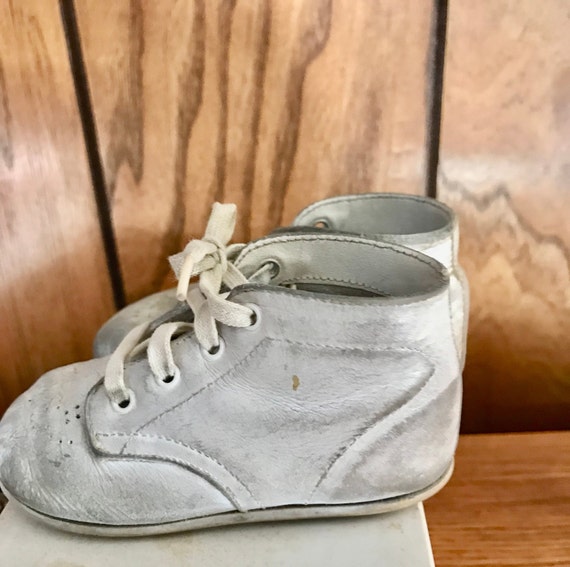This photograph features a pair of vintage baby shoes displayed prominently against a blurred wood-paneled background. The shoes rest atop a white platform, possibly a shoebox, placed on what appears to be a wooden table. Both shoes are predominantly white, showing significant signs of wear including visible creasing, scuffs, and dark spots, indicating they have been well-loved and perhaps stored away for some time. The shoes are made of leather, and each has white shoestrings threaded through four eyelets. The left shoe is more visible, while the right shoe peeks from behind, revealing only its top, back, and a bit of the front. The image captures the nostalgic essence of these small, well-worn artifacts, paying tribute to their history and the tiny feet they once adorned.